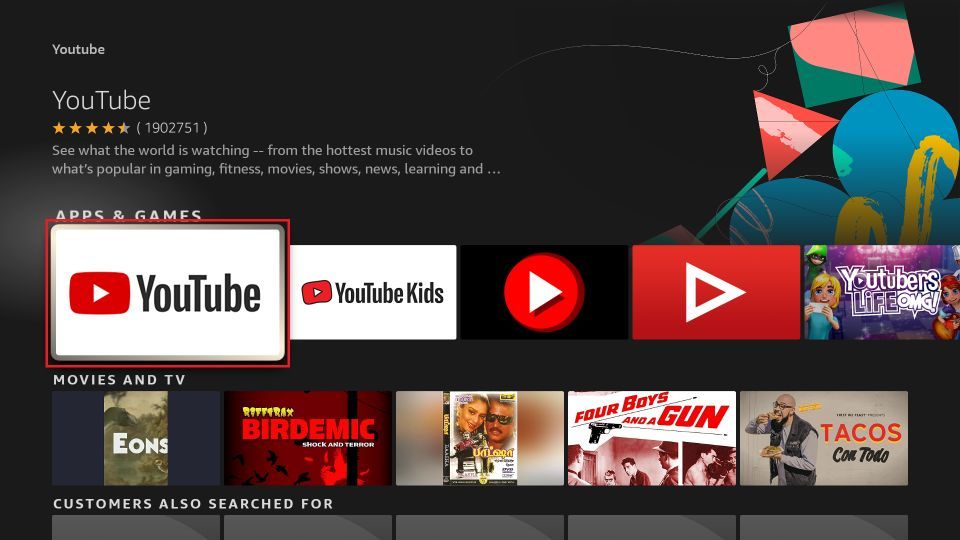### Detailed Descriptive Caption

The image depicts a web page with a black background and various visual elements prominently displayed. In the top left corner, there is the iconic YouTube logo, featuring a capital "Y." Below this, in large white letters, "YouTube" is written again, with a capital "Y" and a capital "T." Adjacent to this text, there is a rating of four and a half stars in orange, followed by the number "902,751" in parentheses. Below the rating, in white type, the text reads: "See what the world is watching – from the hottest music videos to what's popular in gaming, fitness, movies, shows, news, learning, and..."

Below this summary, a heading in all capital white letters says "APPS & GAMES." An orange-bordered rectangle prominently displays the YouTube logo, characterized by a red box with a white play arrow inside and the text "YouTube" with capitalized "Y" and "T." This rectangle appears to overlap slightly with the "APPS & GAMES" heading.

To the right of the YouTube logo, the text "YouTube Kids" appears with a space between "YouTube" and "Kids," which has a capital "K." The "Kids" part shows a similar logo but angled, featuring the red box and white arrow.

Further to the right, the design includes varied visual elements against a black background. There’s a red circle with a white play arrow, and a larger rectangle in red with a similar white arrow pointing right. Another element to the left shows a cartoon girl with blonde hair, wearing a green elf-like hat. Adjacent to her, the text reads "Youtubers" in white with a capital "Y," and below it, "LIFE OMG!" in purple with capital letters, stylized with an exclamation point and a decorative arrow under the "M."

To the bottom of the image, there is a section titled "MOVIES & TV" in all white capital letters, followed by five rectangular advertisements. The first ad is in black and white showing an erupting volcano with the text "EONS" in capital letters. The second ad displays the word "BIRDEMIC" in capital letters on a red background, with additional white text underneath. The third ad features a couple, possibly at a wedding; the woman wears a headdress, and the man has dark glasses and a mustache. The fourth ad has the text "FOR BOYS" written diagonally in red caps on a white background, featuring a black pistol with an arrow at the gun's muzzle. Above the arrow, small letters "AND A GUN" are written, emphasizing the weapon imagery.

The fifth ad presents a bald man with glasses and a goatee, seemingly eating tacos. He wears a black vest and a gray long-sleeved shirt. Next to him, the word "TACOS" is written in large red letters, with cursive text below reading "CON TOBO."

On the left side, a white capitalized text reads "CUSTOMERS ALSO SEARCHED FOR," which is followed by the very top parts of five gray boxes, not fully visible.

This detailed description outlines the busy, colorful composition of the web page, hinting at a vibrant interface designed to attract and engage viewers.